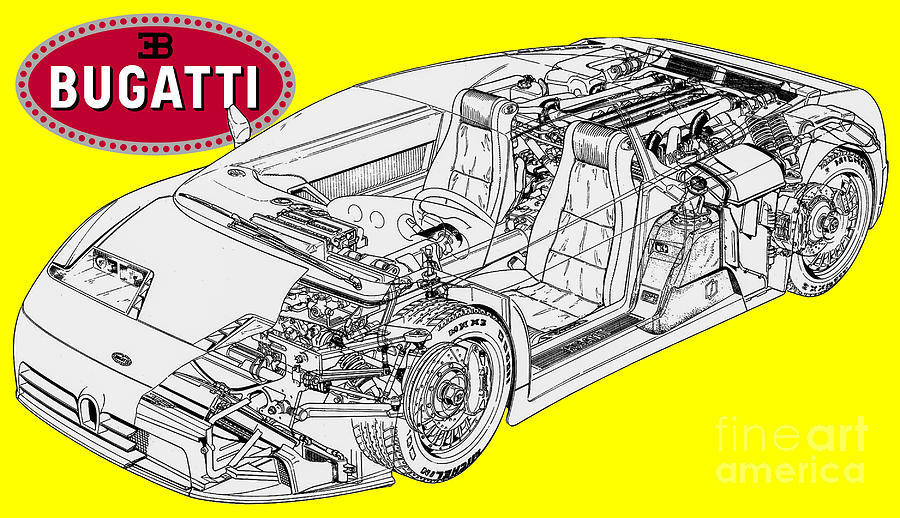The image is a rectangular illustration that's wider than it is tall, featuring a bright yellow background. In the top left corner, there's a gray-bordered, reddish-pink oval logo with white font spelling "Bugatti" and a distinctive emblem above, resembling a connected '3' and 'B'. The artwork presents an intricate, black and white, fine-lined drawing of a Bugatti car, showcasing an exploded view of its inner mechanics. The diagonal perspective reveals detailed components such as the engine and steering mechanisms, with the car's front half opened to expose its internal workings. There are no additional labels or text within the car's drawing, emphasizing the precise and technical artistry involved. Fine Art America is mentioned in the bottom right corner, indicating the piece’s artistic origin.